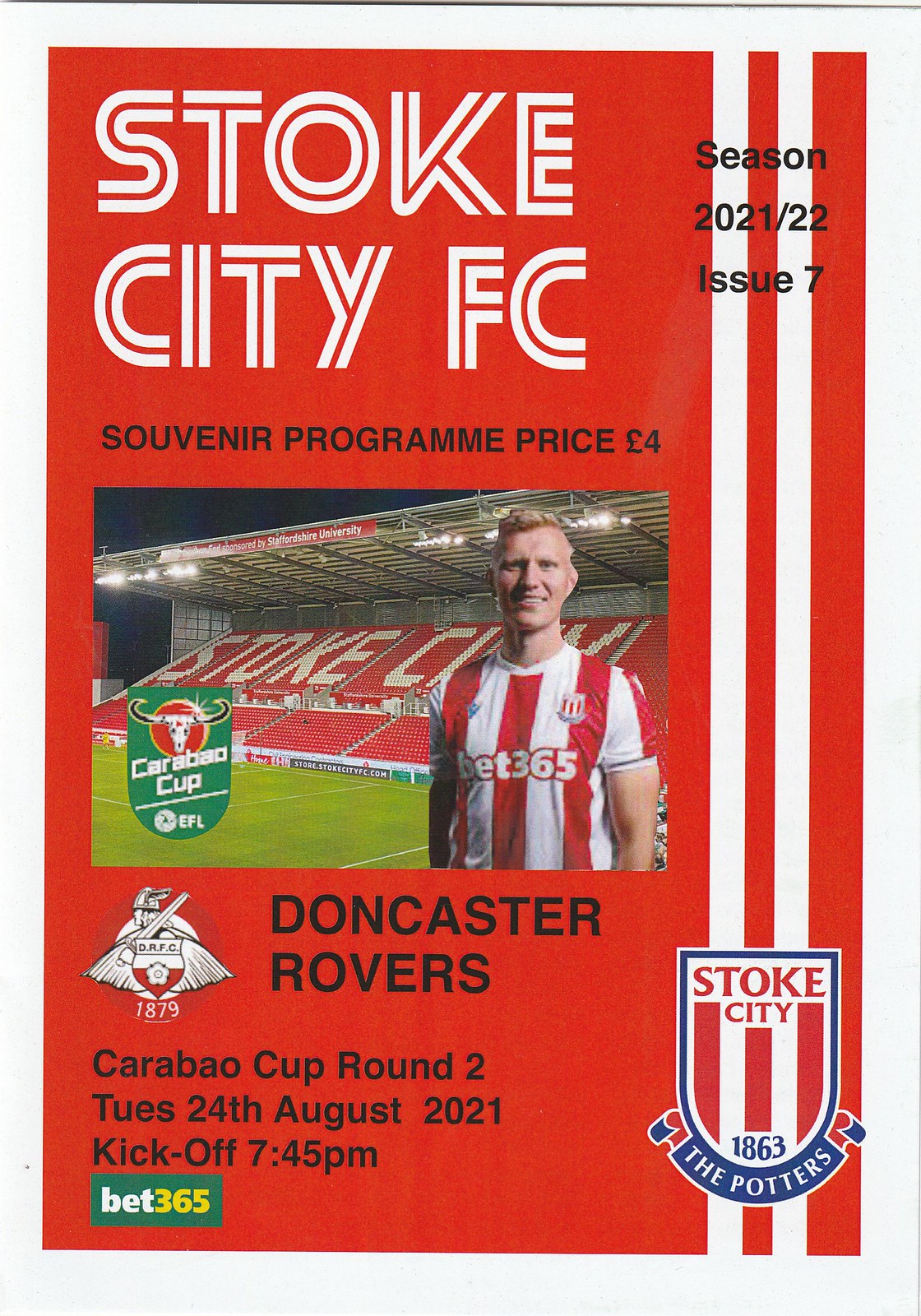The image is the front cover of a magazine or booklet with a tall, vertically aligned rectangular shape and a solid red background. Two thick white vertical stripes run down the right-hand side. In the upper right corner over these stripes, black text reads, "Season 2021/22, Issue 7." 

The title "Stoke City FC" dominates the left side in thick white capital letters, with "Souvenir Program, Price £4" printed in black capital letters below it. A rectangular picture of a man in a vertically striped red and white jersey, which features the text "Bet 365," is prominently displayed in the center. He is standing on a soccer field, with red stands in the background, spelling out "Stoke City" in white letters.

Underneath this picture, the opponent "Doncaster Rovers" is written in all-capital black letters. The bottom of the cover is aligned with more text: "Carabao Cup Round Two, Tuesday, 24th August, 2021, Kickoff 7.45 p.m." Additionally, there is a shield or insignia at the bottom right corner that reads "Stoke City 1863, The Potters," featuring a design of a man facing left holding a sword and a helmet with wings extending out of a shield.